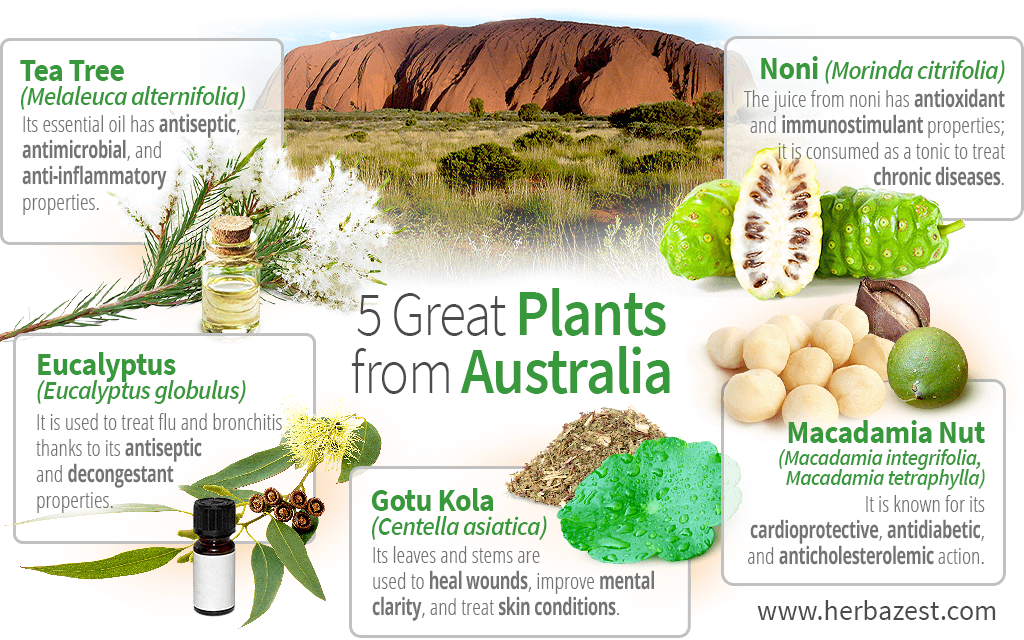The image is an advertisement showcasing "The Five Great Plants of Australia." It features a visually engaging design with a green color scheme highlighting the natural aspect of the plants. At the top, a picturesque scene with a brown mountain and green plains sets an Australian backdrop. Surrounding the central title, there are five informational boxes, each dedicated to a specific plant.

1. **Tea Tree**: The top left box features a tea tree branch with white-tipped leaves and a green stem, as well as a small bottle of essential oil. The text details its antiseptic, anti-microbial, and anti-inflammatory properties.

2. **Eucalyptus**: The next box includes an image of green leaves with black berries, identifying it as eucalyptus. It highlights the plant's use in treating flu and bronchitis due to its antiseptic and decongestant properties.

3. **Gotu Kola**: This box displays a circular green leaf with a brownish ground substance behind it. The accompanying text explains that its leaves and stems can heal wounds, improve mental clarity, and treat skin conditions.

4. **Macadamia Nut**: The fourth box shows an image resembling eggs and a kiwi. It points out the nut's cardioprotective, anti-diabetic, and anti-cholesteric effects.

5. **Noni**: The final box has a picture of a greenish fruit cut open to reveal multiple seeds. It describes noni juice as having antioxidant and immunostimulant properties, consumed as a tonic to treat chronic diseases.

Below these descriptions, the URL www.herbizest.com is displayed for further information.